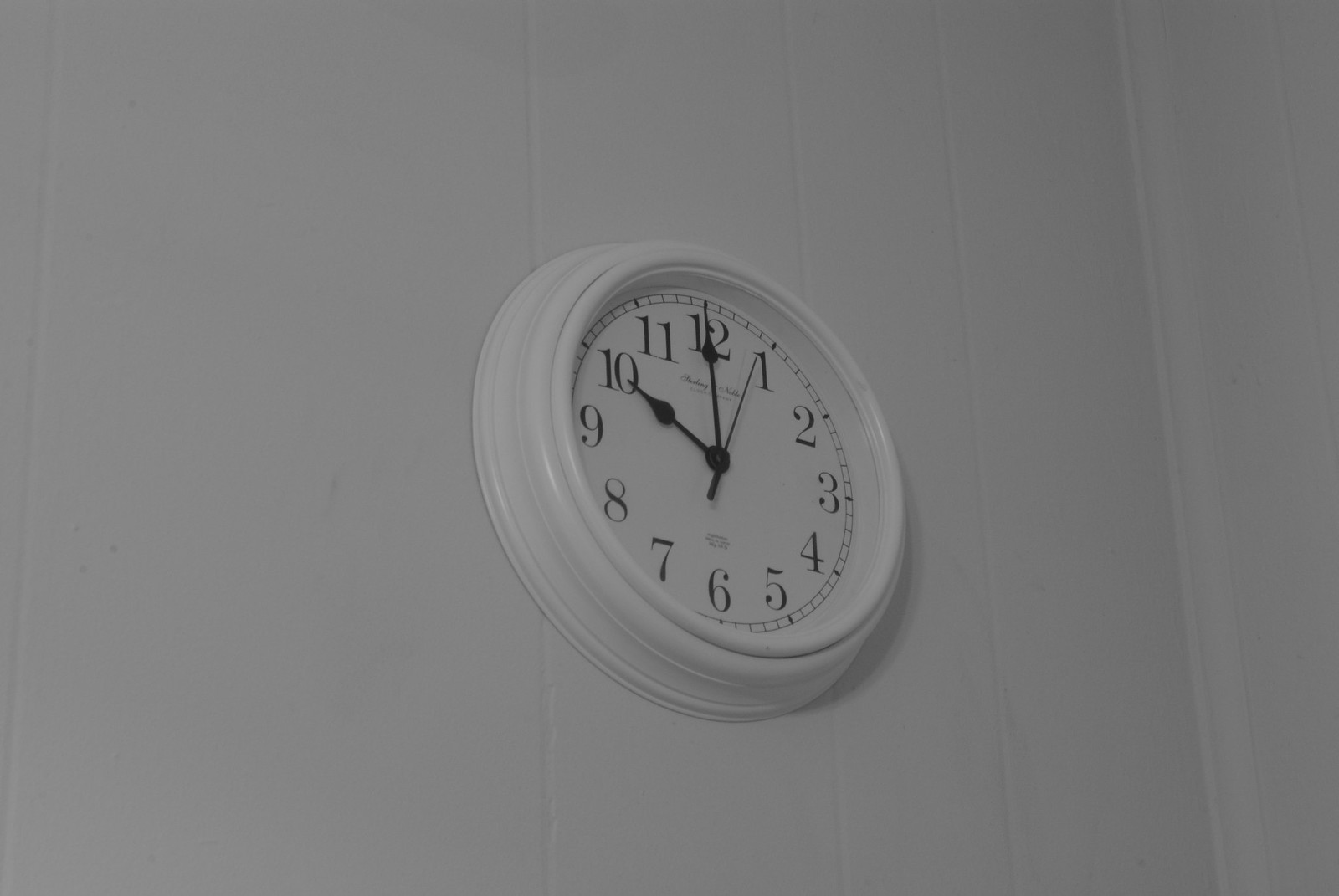The photograph depicts a simple, rectangular image of a wall clock, positioned near the corner where two white walls converge, roughly 10% from the right edge of the frame. The clock, which is slightly angled to the right, features a fairly thick, plastic frame with a design that narrows towards the center, creating a concentric circle effect. The clock's face is white, displaying black Arabic numerals from 1 to 12, each separated by four minute markers. The hour and minute hands, both black and arrow-shaped, indicate the time as precisely 10:00. A long, thin second hand, also black, points one notch short of the 1, suggesting it is about four seconds past 10:00. Though the clock body and wall appear grayish due to lighting or reproduction, they are intended to be white. The image does not reveal any ceiling or elements below the clock.